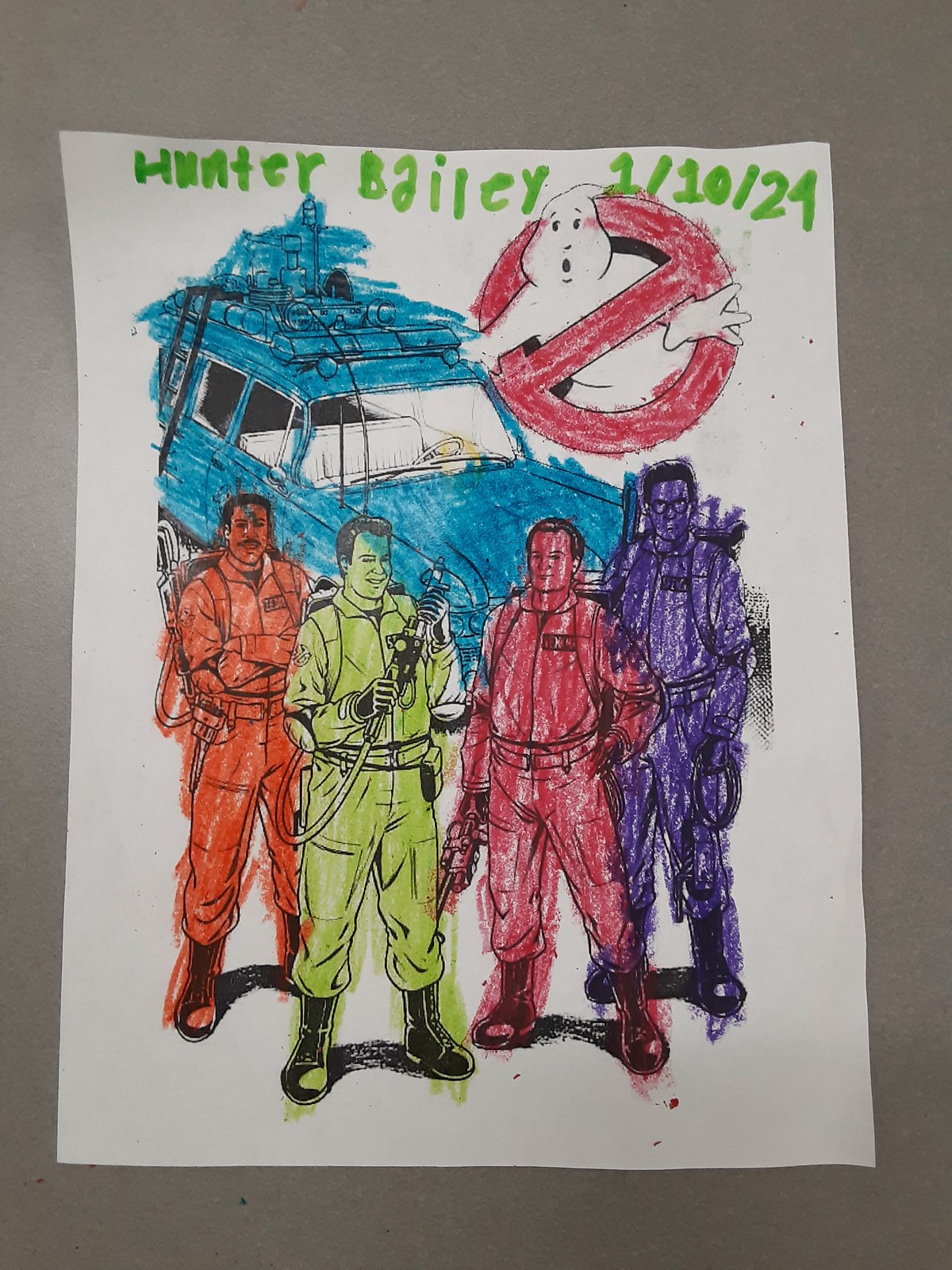This image depicts a child’s crayon-colored illustration of the original Ghostbusters, signed "Hunter Bailey 11024" in green marker at the top. The drawing features four Ghostbusters in front of the iconic Ghostbusters station wagon, with detailed ghost-hunting equipment on the vehicle’s roof. The car is shaded turquoise, with white elements preserved inside. The Ghostbusters logo, prominently located in the upper right corner, showcases the white ghost outlined by a striking red prohibition symbol. Each Ghostbuster is distinctly colored: the one on the far left in orange, followed by green, next in red, and the far right in purple. The crayon texture is evident throughout, indicating the illustration was colored with great enthusiasm, likely by a young fan. The scene is placed against a stark white background, emphasizing the vibrant hues and the playful creativity of the artist.